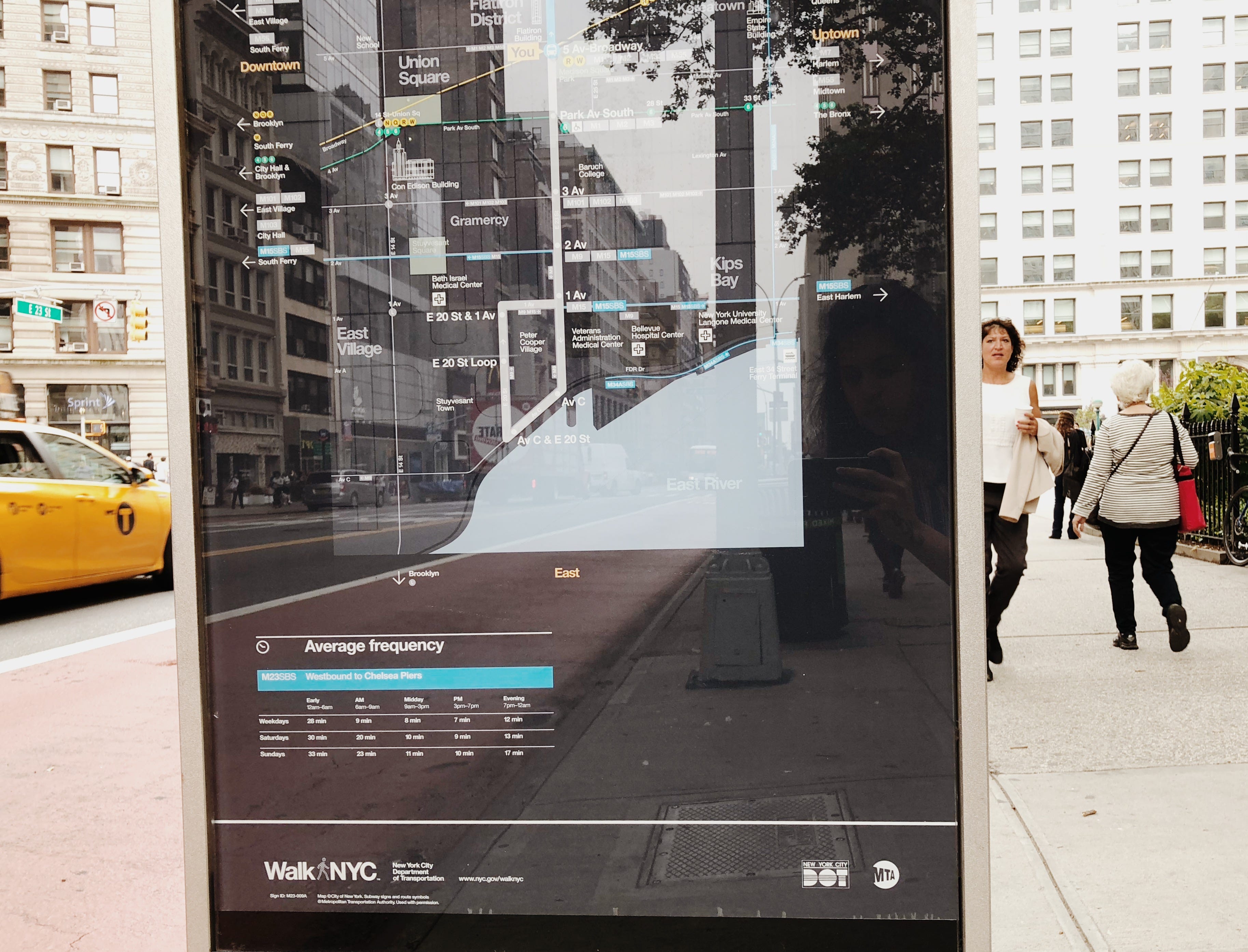The image showcases a close-up of a large kiosk with a translucent glass screen, resembling a giant tablet. The screen vividly displays a detailed map of the city, perfectly mirroring the actual cityscape in the background. The interactive map highlights various sections across the city, pinpointing the viewer's current location and other key areas. Below the screen, the label "WOC NYC" is prominently visible. Towering skyscrapers flank the kiosk on both sides, adding to the immersive urban atmosphere. Within the translucent screen, reflections reveal the photographer holding a cell phone to capture the scene. Further to the right, in the background, two pedestrians are seen walking along the sidewalk, contributing to the bustling city environment.